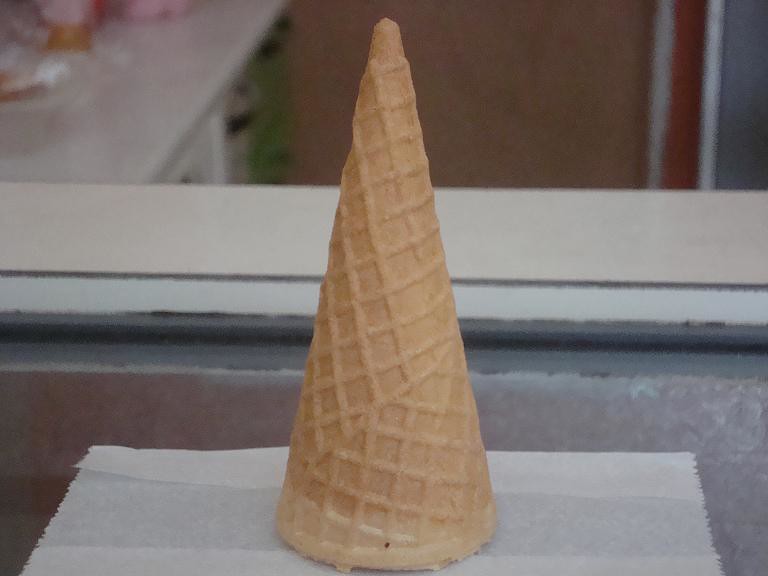The image depicts an empty waffle ice cream cone standing upright with its pointed end on a piece of rectangular, white parchment paper on an L-shaped white counter. The cone is prominently displayed, seeming to be part of a showcase, possibly in an ice cream shop. The background and the counter appear slightly blurry, emphasizing the cone itself. The scene suggests this could be a demonstration of the type of cone used for serving ice cream to customers.